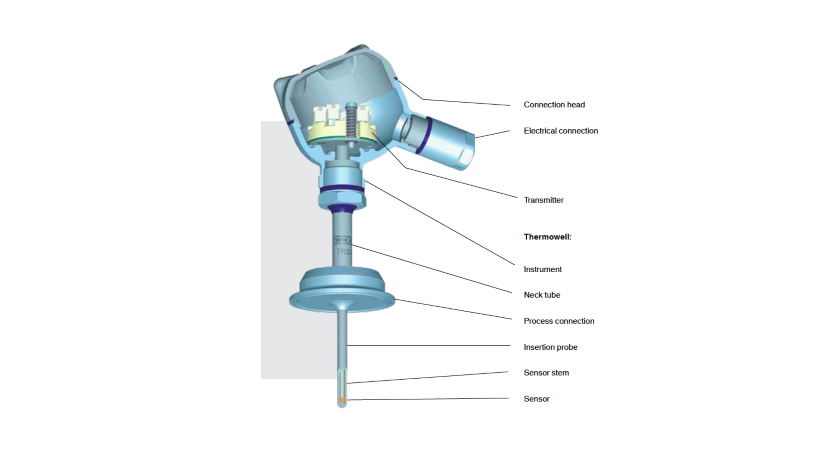The image showcases a detailed diagram of a mechanical device, predominantly light blue in color, which appears to be instructional in nature, similar to those found in manuals or textbooks. The device features a bulbous, circular head at the top with an attached small arm or eyepiece extending from the right side. Below this head, a longer neck or cylinder extends downwards, leading into a segmented pole that progresses vertically. The diagram offers a partly transparent view into the interior components of the equipment, emphasizing its various internal and external parts.

On the right side of the image, black text labels each component of the device with corresponding lines pointing to specific parts. From top to bottom, these labels indicate: Connection Head, Electrical Connection, Transmitter, Thermowell, Instrument, Neck Tube, Process Connection, Insertion Probe, Sensor Stem, and finally Sensor at the bottom. This diagram provides a comprehensive breakdown of the componentry and structure of the device, making it clear and informative for instructional or educational purposes.